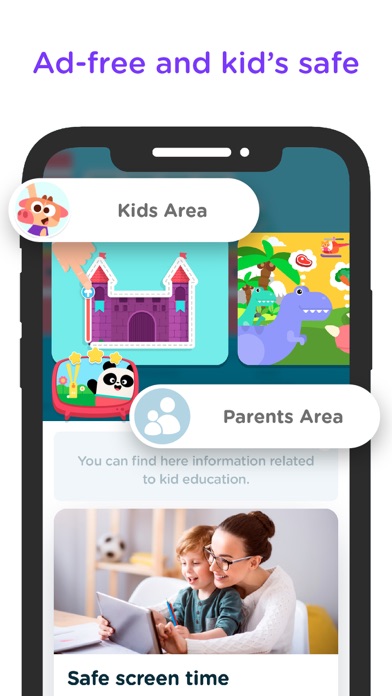The image is an advertisement featuring a mobile application tailored for children and their parents. It starts with a white background, prominently displaying the phrase "Ad Free and Kids Safe" in purple text at the top. 

A partially visible smartphone dominates the central part of the image, with the phone's screen showcasing various features of the app. The upper portion of the phone screen includes a white button on the left side, adorned with an animated character—a pig with a brownish face, large eyes, and wearing a purple shirt. Adjacent to this character, the text "Kids Area" is clearly displayed.

On the phone screen below this, two distinct images are visible. On the left, there is a picture of a purple castle with red turrets, being touched by a hand. The right side image is slightly cut off but features a purple dinosaur, a green dinosaur, palm trees in the background, and a helicopter in the sky. 

Beneath these images, towards the left, there is an illustration of a panda bear and a yellow rabbit. To the right of this is another white button labeled "Parents Area." Below this button, the text explains that it provides information related to children's education. This section is complemented by a photo of a smiling mother and her son sitting on a chair, both engaged with a laptop, their hands touching the device.

At the bottom of the advertisement, the caption "Safe Screen Time" reassures viewers about the app’s safety.